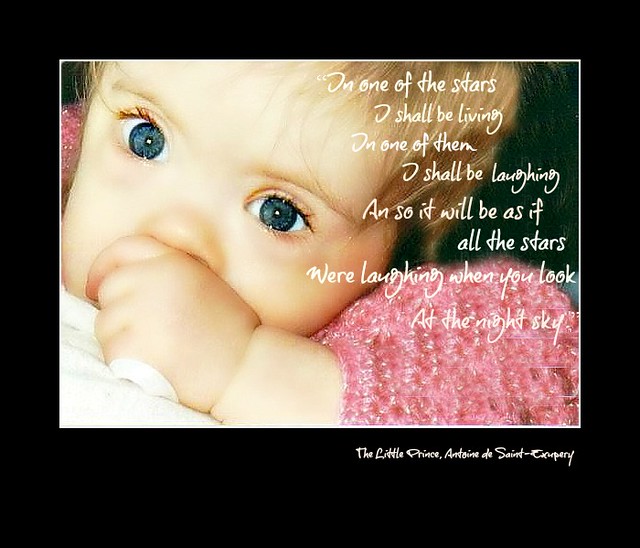This image appears to be an artistic advertisement, possibly for a photography tutor, featuring a close-up of a young baby with smooth white skin, big dark blue eyes, and blonde hair and eyebrows. The baby is wearing a fluffy, shiny pink sweater, and their left hand is partially covering their nose and mouth while their eyes are open wide. The background of the image is stark black, creating a striking contrast. Surrounding the main picture is a white border, which itself is enclosed by a thicker black border. At the bottom of the photograph, in a neat and somewhat difficult-to-read font, it says "The Little Prince, Antoine de Saint-Exupery." Overlaying the image, in white cursive text, is a quote from "The Little Prince" enclosed in double quotes: "On one of the stars I shall be living, on one of them I shall be laughing. And so it will be as if all the stars were laughing when you look at the night sky."